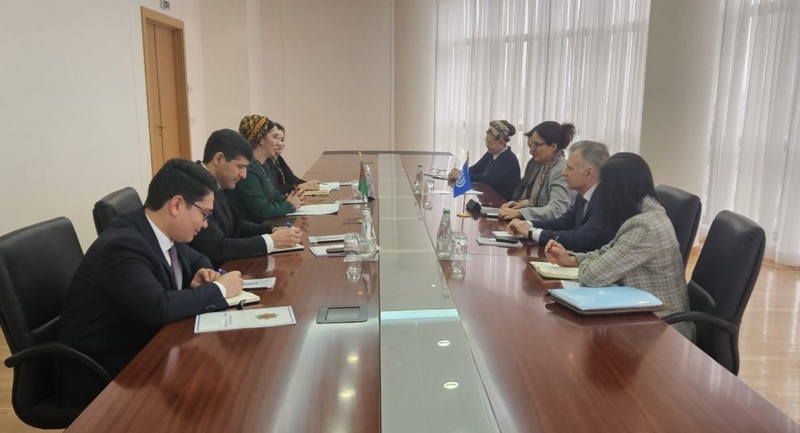This horizontal photograph captures a professional meeting taking place in a well-lit boardroom dominated by a sleek, cherry oak-colored table with a prominent white stripe running down its length. Seated around this long table, which stretches the entire width of the image, are eight individuals, four on each side, all engaged in the session and seated in executive leather chairs. On the left side, two men in suits diligently take notes, one of whom has a certificate in front of him, while further along the table sits a woman in a green long-sleeve jacket adorned with a distinctive yellow and black hat, leading the conversation. Beside her is another person wearing black, whose face is partially obscured. On the right side, the first person in a plaid gray jacket with longer hair faces away from the camera, followed by a man in a suit with gray hair, a woman with glasses and a gray top, and a final individual with a hat, unidentifiable by gender. Various papers, notebooks, plastic drinks, and several country flags, including a blue one, are scattered across the table. The room’s beige walls are complemented by white curtains over the windows, flooding the space with light, and a tan, wood-colored door is visible, hinting at either an exit or an elevator. The atmosphere is lively, with many participants smiling and deeply engaged in conversation.